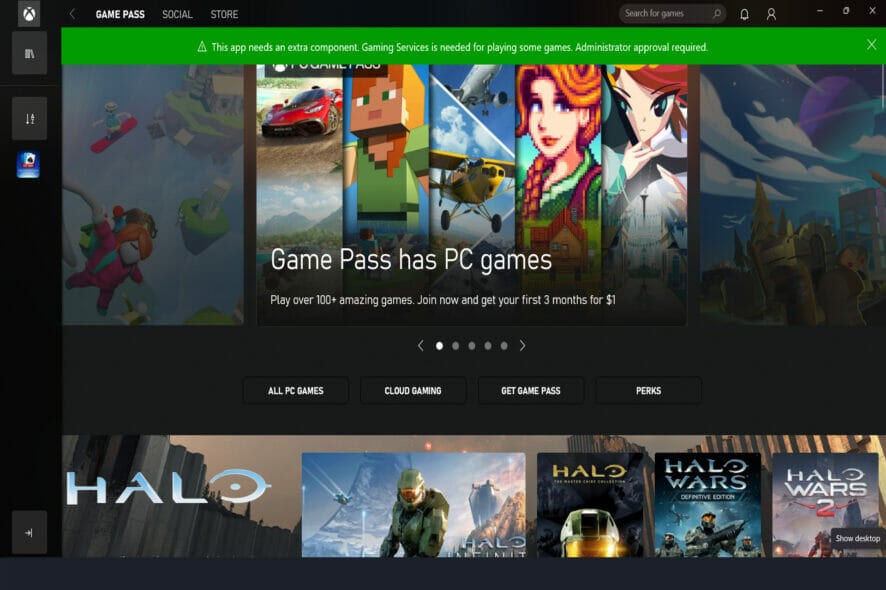The screenshot appears to be of an Xbox interface, likely from the Xbox app or Xbox Game Pass. The background is predominantly black, emphasizing the foreground elements. In the top left corner, there's a recognizable Xbox symbol, confirming the platform. 

Across the top of the screen are several tabs such as "Game Pass" and "Social," which seem to offer different functionalities. "Social" presumably allows users to interact with other players, while "Store" might facilitate game purchases. 

On the right side, there are additional icons possibly related to the user's account settings, including an avatar image depicting a person. A prominent message is displayed indicating that "this app needs an extra component; gaming services required for playing some games" and mentions that "administrator approval" is necessary. 

The central part of the screen showcases several game titles available on Xbox Game Pass. In particular, multiple entries from the Halo series are visible, such as "Halo" and "Halo Wars." Other game genres are represented as well, including an anime-styled game, a racing game, a flight simulation game with an airplane, and a game featuring a Lego character.

Overall, this interface seems to be the main hub or entrance page for accessing a variety of video games available on the Xbox platform.